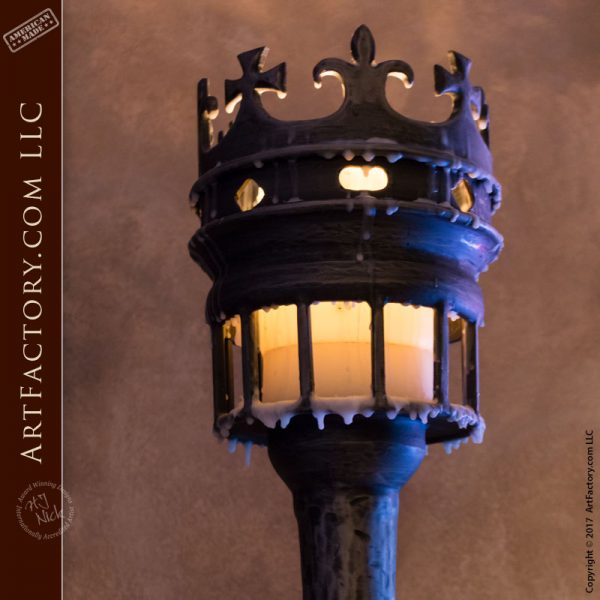The image depicts a highly detailed, close-up view of a medieval English royal-themed torch lamp crafted from metal. The lamp's design features a cylindrical base, transitioning into a tall, black pole. At the top, it culminates in an ornate crown-like structure with cross shapes, prongs, and various intricate symbols, including yellow ovals and teardrop shapes. The centerpiece of the lamp appears to be a lantern or candle with a yellowish-orange glow surrounded by white drippings on a white circle. The entire piece is encased in a round cylindrical cage made of black bars. The background is brown, and the left-hand side prominently displays the text "Artfactory.com, LLC" in beige letters on a maroon background, along with the labels "American-Made" in the top-left corner and "Copyright 2017 Artfactory.com, LLC" in the bottom-right corner. The image is bright and well-lit, showcasing the detailed craftsmanship of the torch lamp.